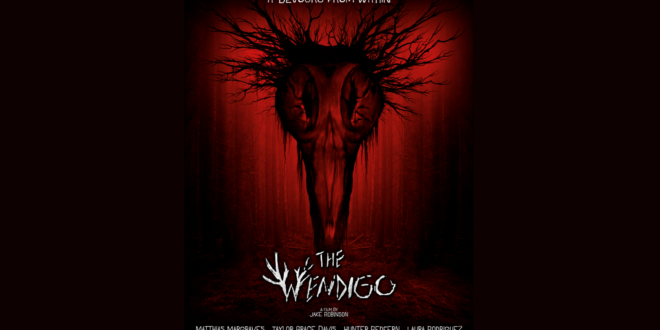The image is a narrow, horizontal poster, predominantly black with a dark, eerie atmosphere. At the center is a heart-shaped burst of red light, illuminating a terrifying creature. This creature has a rounded, light bulb-shaped head adorned with tree branch-like appendages that resemble hair. Its eyes are narrow, snake-like, and deeply set, giving a haunting look alongside the long, beak-like protrusion extending from its face. The creature's sinister appearance suggests it is the Wendigo. Below the creature's head, in white uppercase letters with tree branches intertwined in the 'W,' is the title, "THE WENDIGO." Just beneath the title, the caption reads, "A film by Jake Robinson," though some additional text below is partly obscured. The names of the actors, including Taylor Grace and a possible Rodriguez, are partially cut off and difficult to discern. The dark, burgundy hues and ominous design elements create a haunting, foreboding visual indicative of a horror film poster.